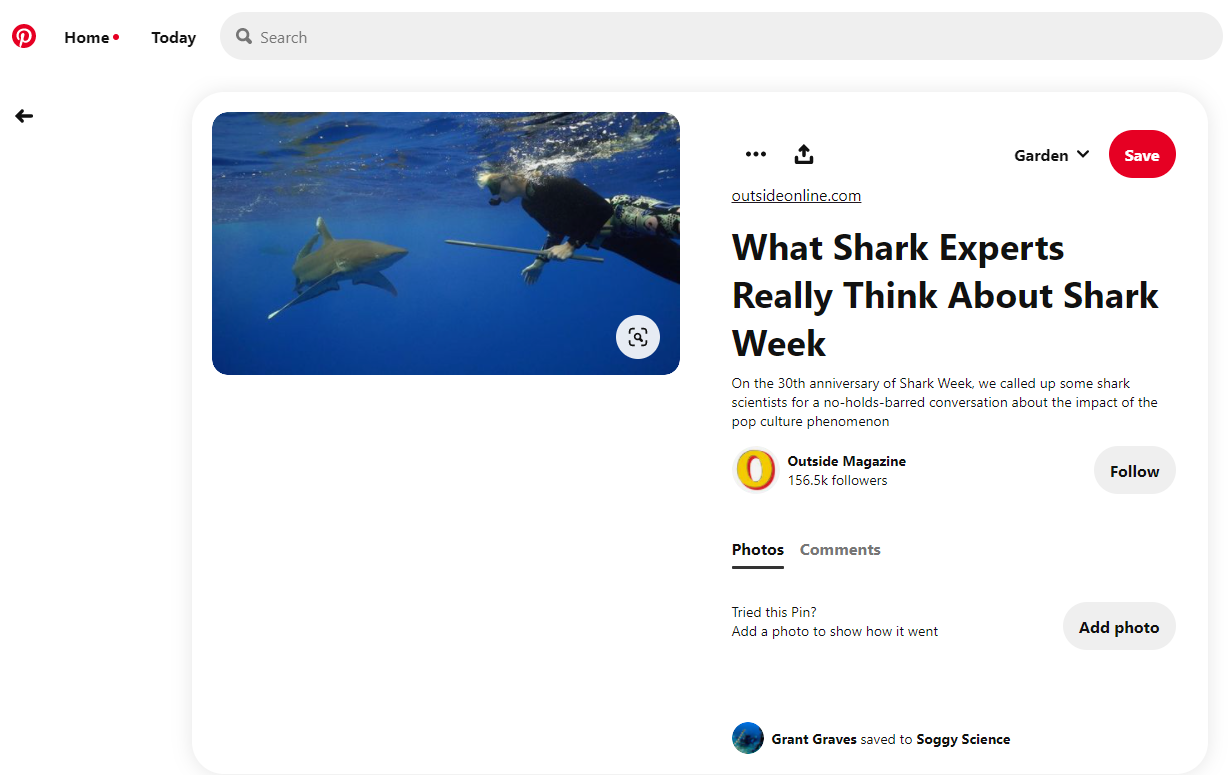In the left-hand side of the image, the vibrant blue waters set a striking backdrop as a solitary gray shark glides through the depths. In the foreground, a scuba diver is captured in action, dressed in a black wetsuit complemented by camo pants, with a bang stick in one hand, indicative of a poised, cautious approach. 

At the top left corner, a prominent red picture symbol catches the eye, accompanied by black text. Adjacent to this symbol is an array of icons including a gray circle with a dot, a dotted square, an upward arrow, and a red object that remains undefined. The text "outsideonline.com" appears, alluding to an article or media content from the site.

The highlighted headline asks, "What do shark experts really think about Shark Week?" In commemoration of Shark Week's 30th anniversary, several shark scientists have been contacted for a candid discussion about the cultural phenomenon's true impact.

Below this, there is a notable 'O' representing Outside Magazine, which boasts a following of 156.5 thousand. A gray circle with black text prompts viewers to "follow" the publication. Additional interactive options are displayed with text reading, “Photos, comments, try this pin? Add a photo to show how it works? No, add photo.”

Lastly, a blue circle profile icon marks the user Grant Graves, who has saved this content to a board named “Soggy Science.” The user’s name, Grant Graves, and the board's title, "Soggy Science," are reiterated to underline the personalized collection of aquatic and scientific interests.